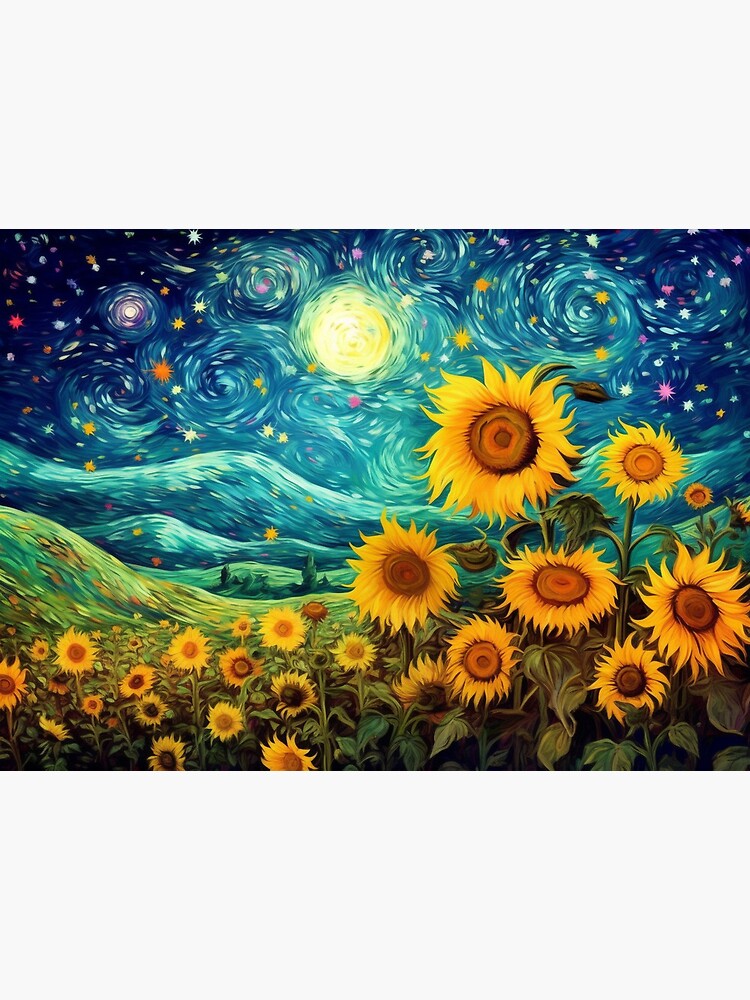This painting, titled "Sunflower Field Under a Starry Night," showcases a vivid Van Gogh-inspired scene. Framed by a wide white border at the top and bottom, the artwork exhibits the characteristic swirling patterns reminiscent of Van Gogh's "Starry Night." The sky is a dynamic swirl of blue, populated by colorful, multi-sized stars—orange, yellow, purple, white, and blue—and a bright moon. Below this celestial dance, rolling green and blue hills undulate like gentle ocean waves. These hills transition into a lush field of sunflowers stretching across the bottom of the image, from left to right. The sunflowers display spiky, wavy petals, with the largest blooms positioned prominently in the bottom right corner, gradually decreasing in size towards the bottom left. The overall composition captures the energy and intensity of Van Gogh's iconic style, merging the serene fields with a vibrant, swirling nighttime sky.